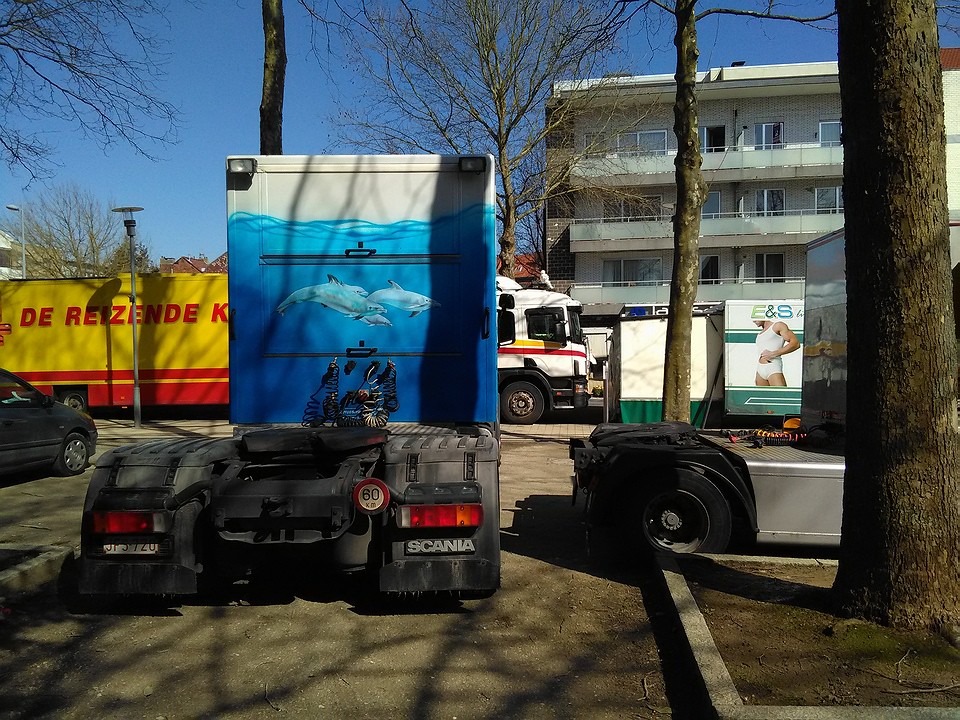The photograph captures a daytime scene in a parking lot outside a motel or possibly a multi-storey building. Dominating the foreground is the cab of a blue truck, distinctively painted with a mural of dolphins frolicking in ocean waves; the top portion of the cab is painted white. Nearby, another truck cab is partially visible, showing just its tires. Also prominent in the image is a large yellow and orange moving van displaying the text "D-R-E-I-Z-E-N-D-E-K" in orange letters, with its cab featuring white along with matching orange and gold stripes. Further behind, a silver truck is partially obscured by a tree planted in a planter box. In the far back, there is a red and yellow truck near apartment buildings, as well as a small black car to the left side. The scene is framed by a blue sky above and a road or another section of the parking lot running horizontally through the middle of the image.